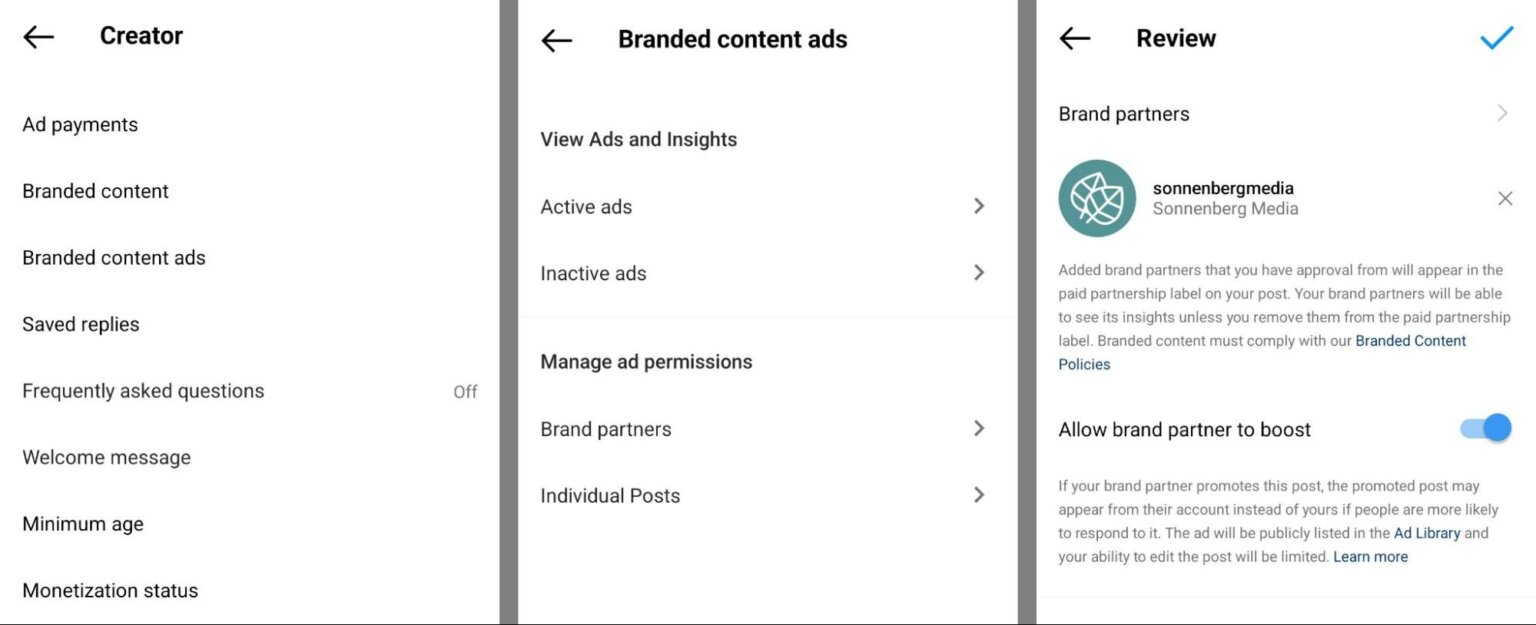The composite image comprises three distinct screenshots that appear to be from a YouTube settings interface or a similar content management system. 

**Left Screenshot:**
The leftmost image is titled "Creator," featuring a back button indicated by an arrow pointing to the left. This section displays various operational tabs for content management and monetization. Listed from top to bottom, the tabs include:
- Add Payments
- Branded Content
- Branded Content Ads
- Saved Replies
- Frequently Asked Questions (currently toggled off)
- Welcome Message
- Minimum Age
- Monetization Status

**Middle Screenshot:**
The central image is specifically focused on the "Branded Content Ads" tab, which is presumably selected from the previously mentioned "Creator" tab. This section is subdivided into several components:
- View Ads and Insights
- Active Ads (with a right arrow indicating more options)
- Inactive Ads (with additional options available)
- Manage Ad Permissions
- Brand Partners
- Individual Posts

**Right Screenshot:**
The rightmost image appears to be a review screen, identifiable by a blue checkmark indicating verification. Within this section, the following options and statuses are visible:
- Brand Partners
- Sonnenberg Media
- An option labeled "Allow Brand Partner to Boost," which is currently toggled on

Overall, these images illustrate different facets of content and ad management within a creator's settings dashboard, including payment setups, ad insights, and brand partnership functionalities.